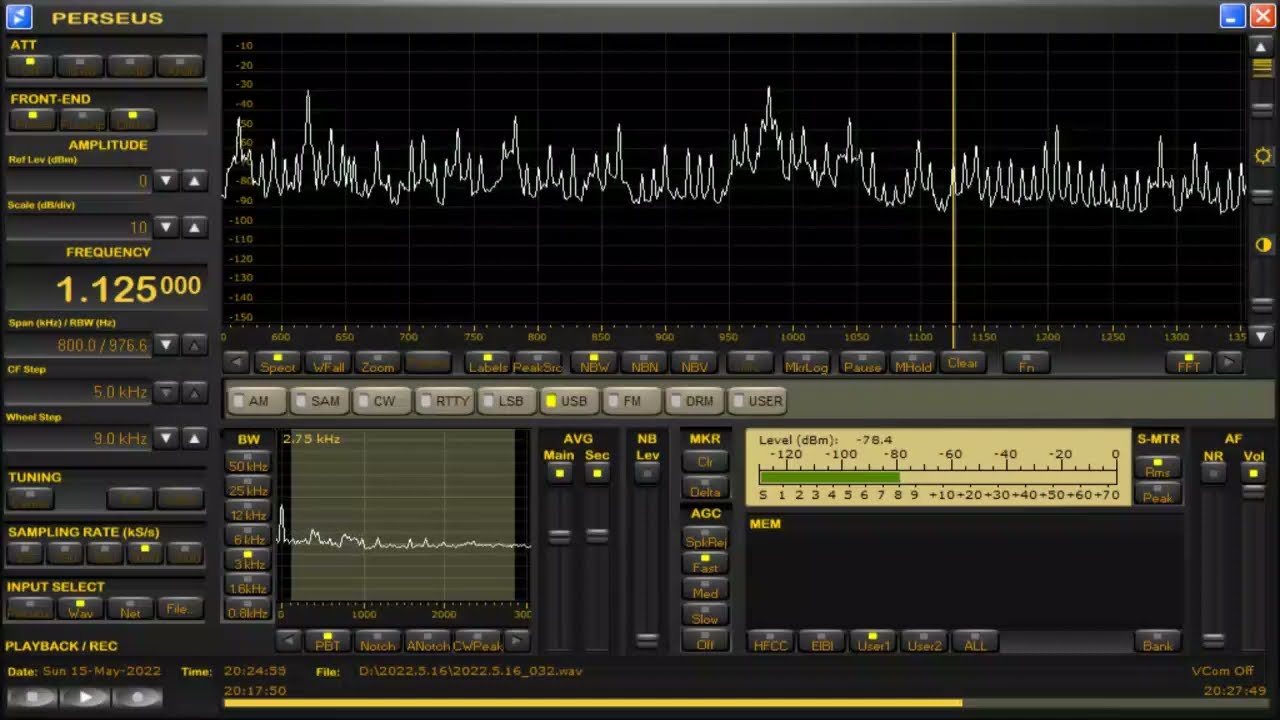The image displays a detailed interface of what appears to be music production or sound mixing software, identified as "PERSEUS" in the top left corner. The application screenshot, likely from a computer, includes the standard window controls: a red square with an X for closing, a blue square with a white dash for minimizing, and a blue square with two opposing arrows for maximizing the window.

On the left side is a vertical panel featuring numerous black buttons with gold text, labeled with terms crucial for audio control, such as "amplitude," "frequency," "sampling rate," "input select," "front end," "playback," "recording," and "tuning." Towards the center top is a broad horizontal panel against a black background, displaying white waveforms reminiscent of an EKG monitor, illustrating real-time sound wave or frequency data.

Below this waveform panel, a series of buttons in different hues are organized. Black buttons with gold writing and light brownish-gold buttons with black text provide various control options. Another smaller waveform display is located in a green box on the lower left, surrounded by additional buttons, which likely allow for detailed adjustments and monitoring.

On the right side at the top, there is a yellow vertical line within the waveform, indicating the current tuning frequency set precisely to 1.125000. Near the bottom right, a decibel meter is present, with a MEM function and green indicators reaching up to -15 on a brown number line background. Red arrows on black buttons suggest functionalities for fine-tuning settings or navigating through different controls.

In summary, this intricate user interface of the "PERSEUS" software is equipped with various visual and interactive elements for detailed audio manipulation and monitoring, emphasizing its use in sound engineering or music production.